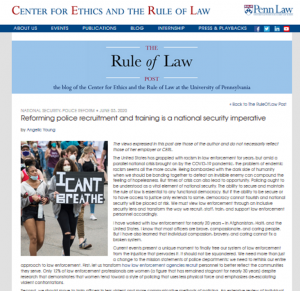The image depicts a webpage from the Center for Ethics and the Rule of Law. At the top of the page, the title "Center for Ethics in the Rule of Law" is prominently displayed, with each word in blue and the capital letters in red. To the right of the title, the logo of Penn Law is visible. Below this, a blue navigation bar is present, although the text within it is too small to be distinguishable.

A large square banner occupies the center of the image, featuring the phrase "The Rule of Law" in bold black letters. The words "The" and "Law" have red accents on the top and bottom, separated by thin white lines on either side. Beneath this banner, the text is too small to read clearly.

The main body of the page features an article titled "Reforming Police Recruitment and Training is a National Security Imperative." The author's name is too small to decipher. Adjacent to the article's title, there is an image of a Black Lives Matter protest, showing people in the streets holding a sign that reads "I Can't Breathe." The paragraph text next to the image is also too small to read.